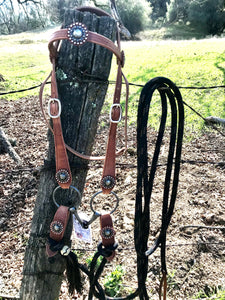This color photograph, captured in portrait orientation, prominently features a dark gray, weathered wooden post, which slants slightly toward the center of the image. The focal point of the photograph is a decorative horse bridle draped over the post. The bridle, crafted from dark brown leather, exhibits artistic detailing with round medallions that boast silver centers surrounded by a bead effect. Multiple straps of the bridle hang along each side, with metal rings at their ends, adding to the intricate composition. Adjacent to the bridle, a dark brown rope lead dangles over the fence wires strung across the post.

In the background, a lush green meadow and a scatter of darker green trees contrast with the muted tones of the post and harness, enriching the natural rustic atmosphere. The overall color palette of the image consists of earthy browns and blacks contrasted by vibrant greens, capturing the serene farm setting. The photograph, characterized by its representational realism, centers on the bridle, suggesting it may hold personal significance or serve as a distinctive ornamental display.